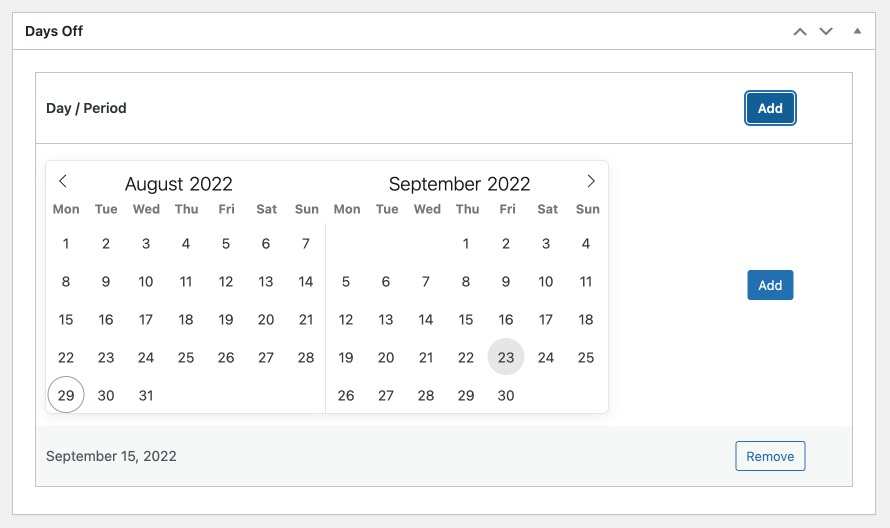The image features a digital calendar layout set against a white background, meticulously outlined in gray. A prominent gray border encases the entire calendar. At the top, a black header reads "Days Off," flanked on the far right by small, up and down arrows for navigation. Directly below, another fine gray line segments the top portion from the rest of the calendar.

Centered beneath this is the label "Day-Period" in black text. Adjacent to this on the right side is a small blue button with a white border, inscribed with the word "Add" in white text.

The main calendar section is divided into two months. On the left, "August 2022" is displayed with a left-pointing arrow next to it. The days of the week—Monday through Sunday—are listed across the top, with the numerical days starting at 1 on Monday and continuing sequentially to 31. Notably, the 29th is circled in gray.

A fine line separates the August calendar from the one for September positioned on the right. Labelled "September 2022," this section also features a right-pointing arrow next to the month name. The days of the week align similarly, beginning on a Thursday with the 1st and proceeding to the 30th. The 23rd is marked distinctively by a shaded circle.

Additionally, another blue "Add" button appears on the right sidebar of the September calendar. At the bottom of the image, a gray-shaded strip spans the width of the calendar. "September 15, 2022" is marked on the left side of this strip, while the far right features a blue-bordered button, filled with white and labeled "Remove" in blue text.